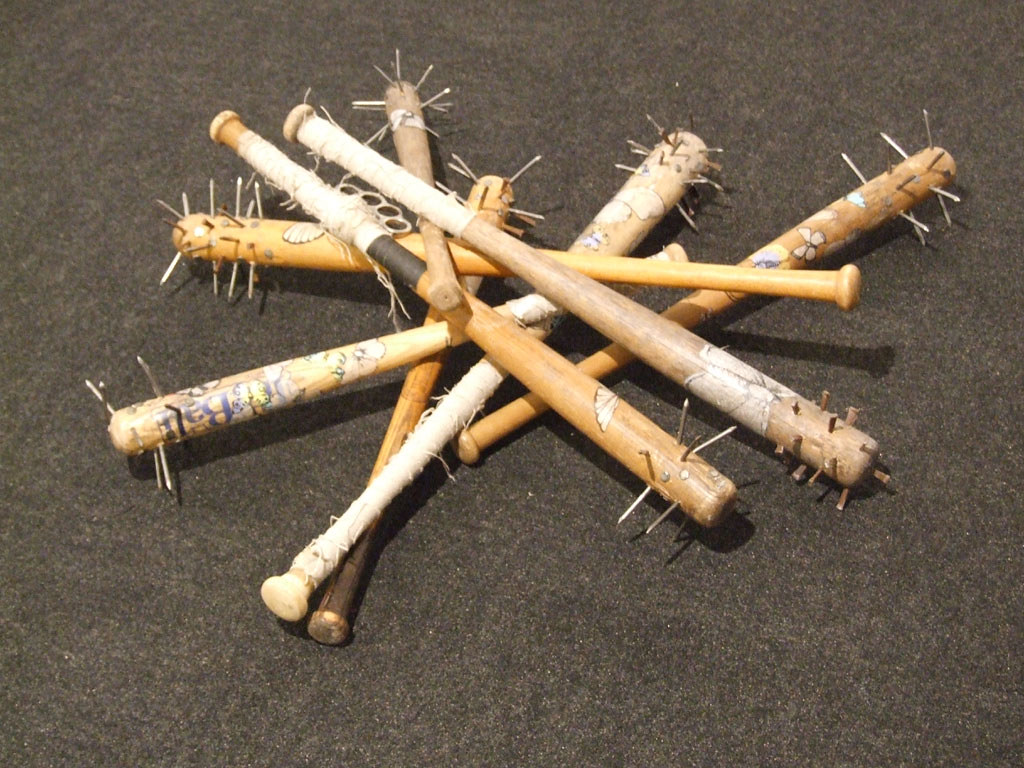The photograph displays a chaotic pile of eight light-colored, wooden baseball bats, crisscrossed in various directions on a dark gray, rough surface. Each bat has been retrofitted with menacing spikes or nails, particularly near the barrel, giving them a dangerous appearance. Some of the nails appear rusty, adding to the distressed and weapon-like aesthetic. The handles of several bats are wrapped in white tape, presumably for grip, while one bat on top is notably adorned with a pair of silver brass knuckles, enhancing its intimidating look. The bats are also decorated with various graffiti-like paintings and stickers, including butterflies and other details, that add a surreal contrast to their otherwise aggressive modifications.